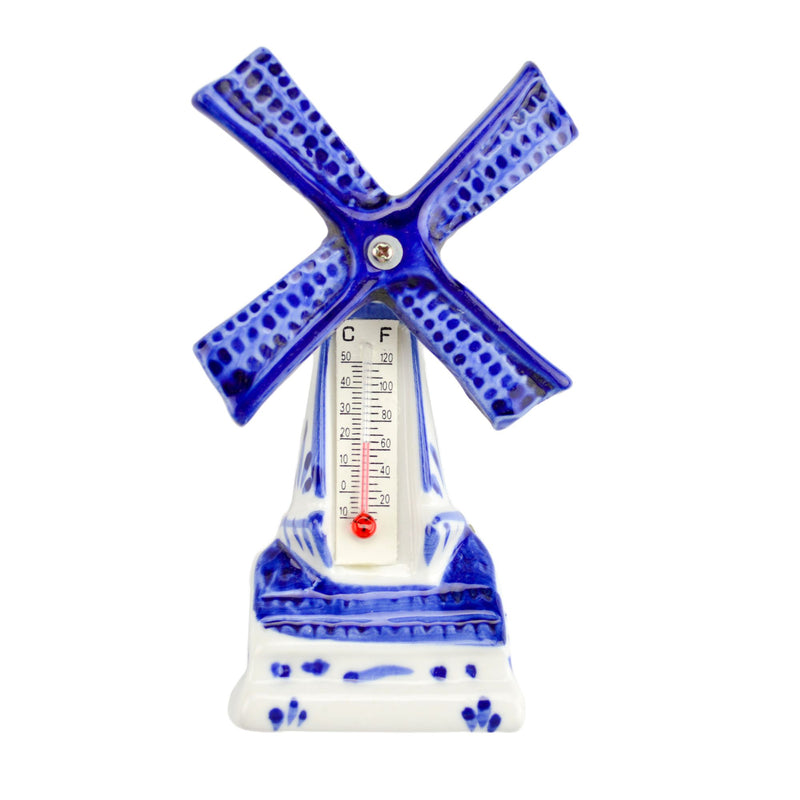This image features a photorealistic thermometer designed in the shape of a windmill. The windmill has four textured blue blades with a silver screw in the center, giving it a distinct pinwheel appearance. The thermometer’s stem, adorned with blue and white designs, contains the actual thermometer. It displays readings in Celsius and Fahrenheit, indicating a temperature of approximately 62-65 degrees Fahrenheit or about 20 degrees Celsius. The base of the windmill is mainly white with blue patterns. The overall construction appears to be made of glass or plastic, with intricate blue and white detailing. The image itself has no border or background color, emphasizing the unique blend of functionality and art.